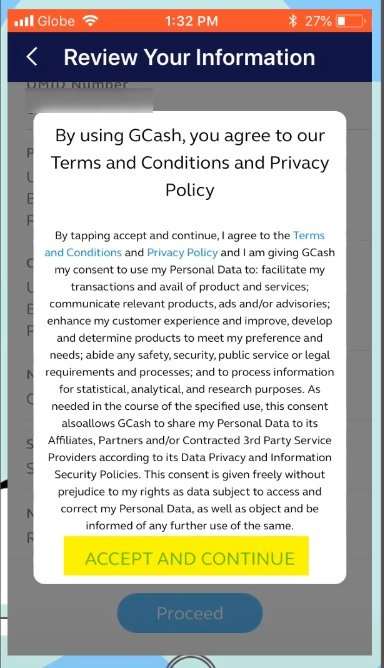This image is a screenshot of an informational page, specifically a privacy policy and terms and conditions agreement for the GCash application. The screenshot is timestamped at 1:32 PM. At the top of the screen, the status bar shows details such as a 27% battery level on the top right and the carrier name "Globe" on the top left. The top section of the screen is orange, which slightly obscures some text, but the heading clearly reads "Review Your Information."

Below the heading, there is a lengthy and detailed explanation of GCash's privacy policy and terms of service. The text elaborates that by tapping "Accept and Continue," the user agrees to the terms and conditions, and consents to allow GCash to use their personal data to facilitate transactions, offer products and services, and communicate relevant products, advertisements, and advisories. Additionally, it states that the user consents to the use of their data to enhance customer experience, improve and develop products to meet preferences and needs, comply with safety, security, public service, or legal requirements, and to process information for statistical, analytical, and research purposes. The consent also allows GCash to share personal data with its affiliates, partners, and third-party service providers in accordance with their data privacy and information security policies.

At the bottom of the screen, there is a prominent yellow button labeled "Accept and Continue."